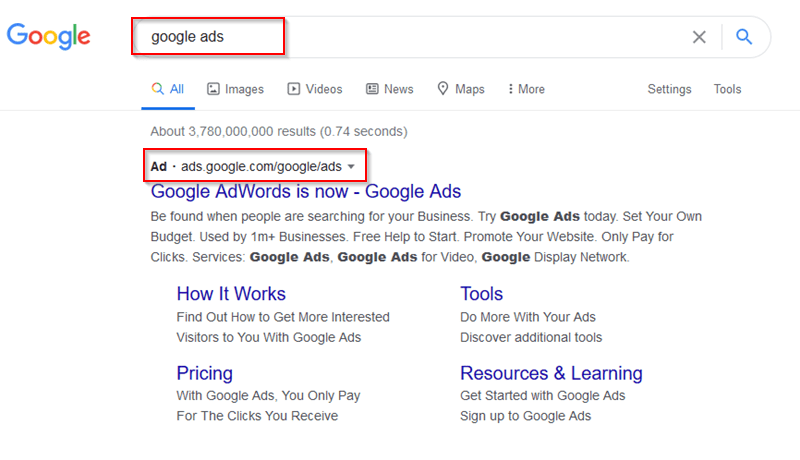The image depicts a Google search page with a search for "Google Ads" highlighted by a prominent red border around the search bar. The iconic Google logo is displayed to the left, with the first 'G', second 'g', and 'l' letters in blue, the first 'o' in red, the second 'o' in yellow, and the 'e' in red. The search query "Google Ads" returns approximately 3,780,000,000 results in just 0.74 seconds.

The central promotional content focuses on Google Ads, encouraging businesses to "Be found when people are searching for your business." The call to action urges users to "Try Google Ads today" and mentions key benefits such as setting your own budget, being used by over 1,000,000 businesses, and offering free help to start and promote your website. Furthermore, it highlights that advertisers only pay for actual clicks.

Below the main promotional text, there are two columns detailing various aspects of Google Ads, each with bold, highlighted subheadings:

1. **How it Works**: Learn how to attract more interested visitors to your business using Google Ads.
2. **Pricing**: Information about paying only for the clicks you receive.
3. **Tools**: Enhance your ads with various tools.
4. **Resources and Learning**: Get started with Google Ads and access resources to enhance your advertising efforts.

Each section provides a brief description to guide users through the benefits and functionalities of using Google Ads for their business needs.